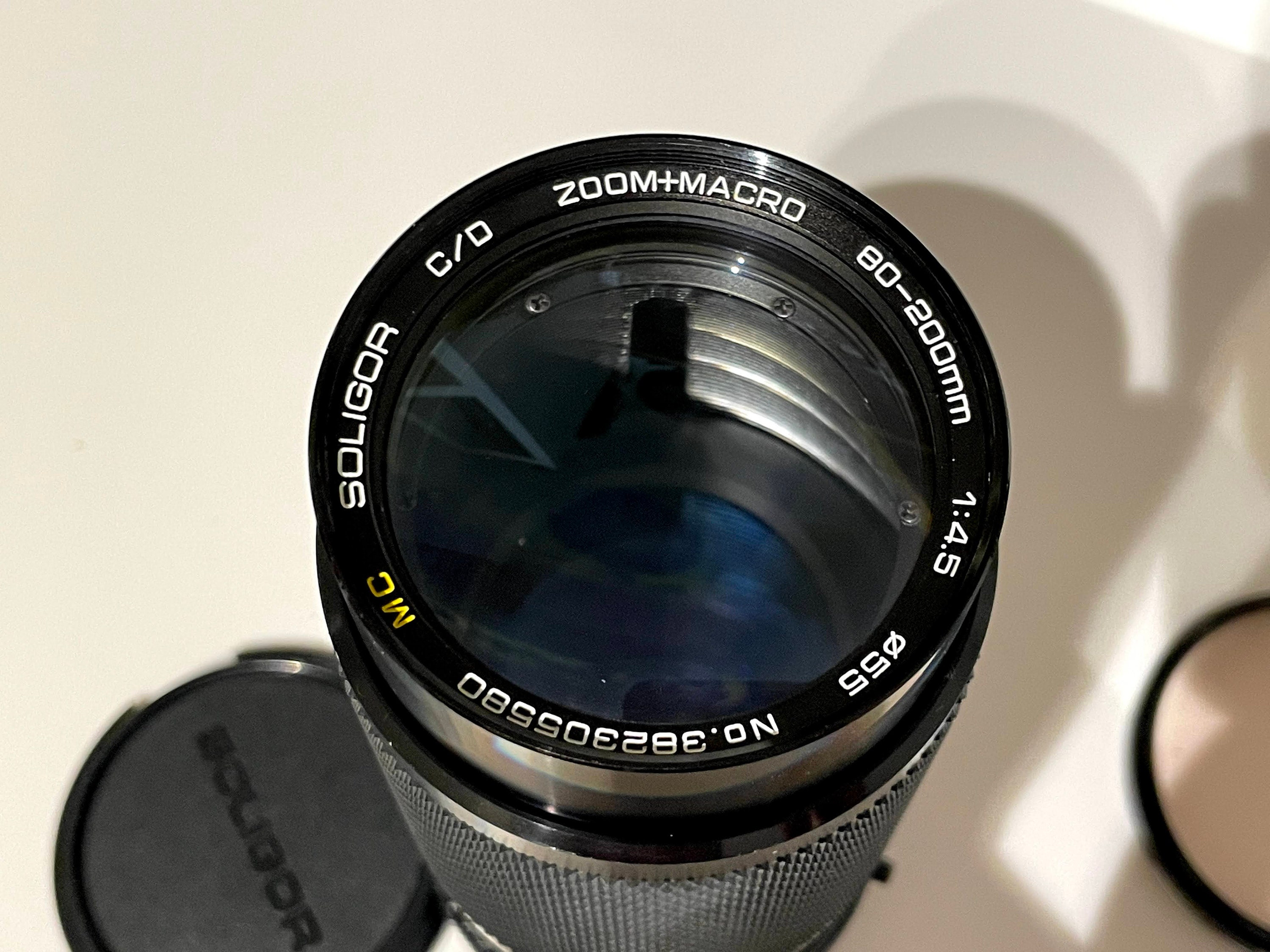This image showcases a Soligor C/D zoom macro camera lens, prominently positioned upright at the center. The lens, black with intricate white text encircling the rim, details its specifications: "Soligor C/D Zoom/Macro 80-200mm, 1:4.5," along with a serial number "382385580" and the notation "MC" in yellow. To the left of the lens, the Soligor-branded lens cap lies on what appears to be an out-of-focus countertop in the background. An intriguing detail reflected in the lens reveals a flip phone, hinting it was used to capture the photograph.